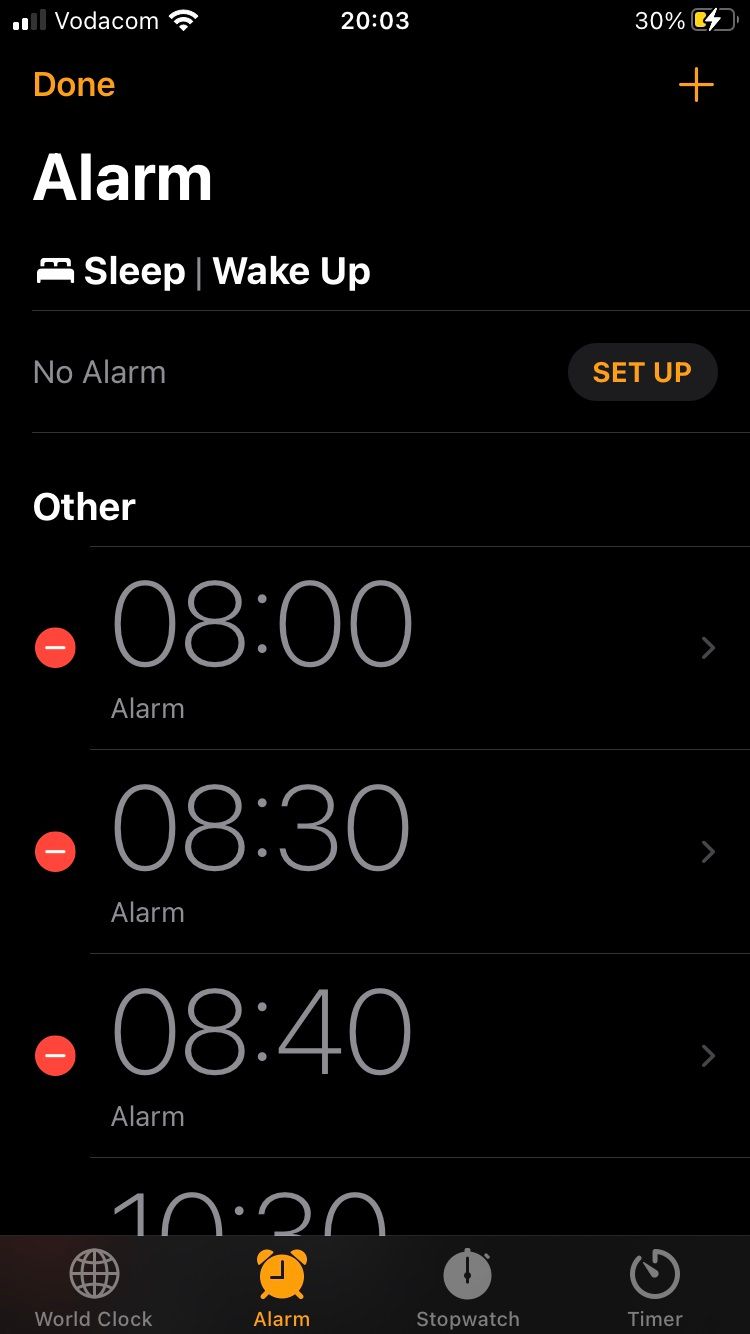A detailed screenshot of a clock app is depicted. At the top, a row of icons indicates phone status, with the signal strength showing two bars and the carrier labeled as Vodacom. Adjacent to it, the Wi-Fi symbol is visible, indicating connectivity. The current time, displayed prominently in the center, reads 20:03. On the left side of the top bar, a battery icon indicates a 30% charge.

Directly beneath the top bar, two buttons are present: "Done" on the right and a plus (+) sign on the left. Below these, the word "Alarm" is displayed, followed by "Sleep/Wake Up."

The screen then notes that no alarms have been set, prompting the user to "Set Up." The entire background is black, providing a clear contrast for the text and icons.

Three alarms are visible, set for 08:00, 08:03, and 08:04 respectively. A fourth alarm set for 10:30 is partially visible at the bottom edge of the screen.

At the bottom of the interface, four tabs offer additional functionalities: World Clock, Alarm, Stopwatch, and Timer, each represented by a simplified icon located just above their respective labels.